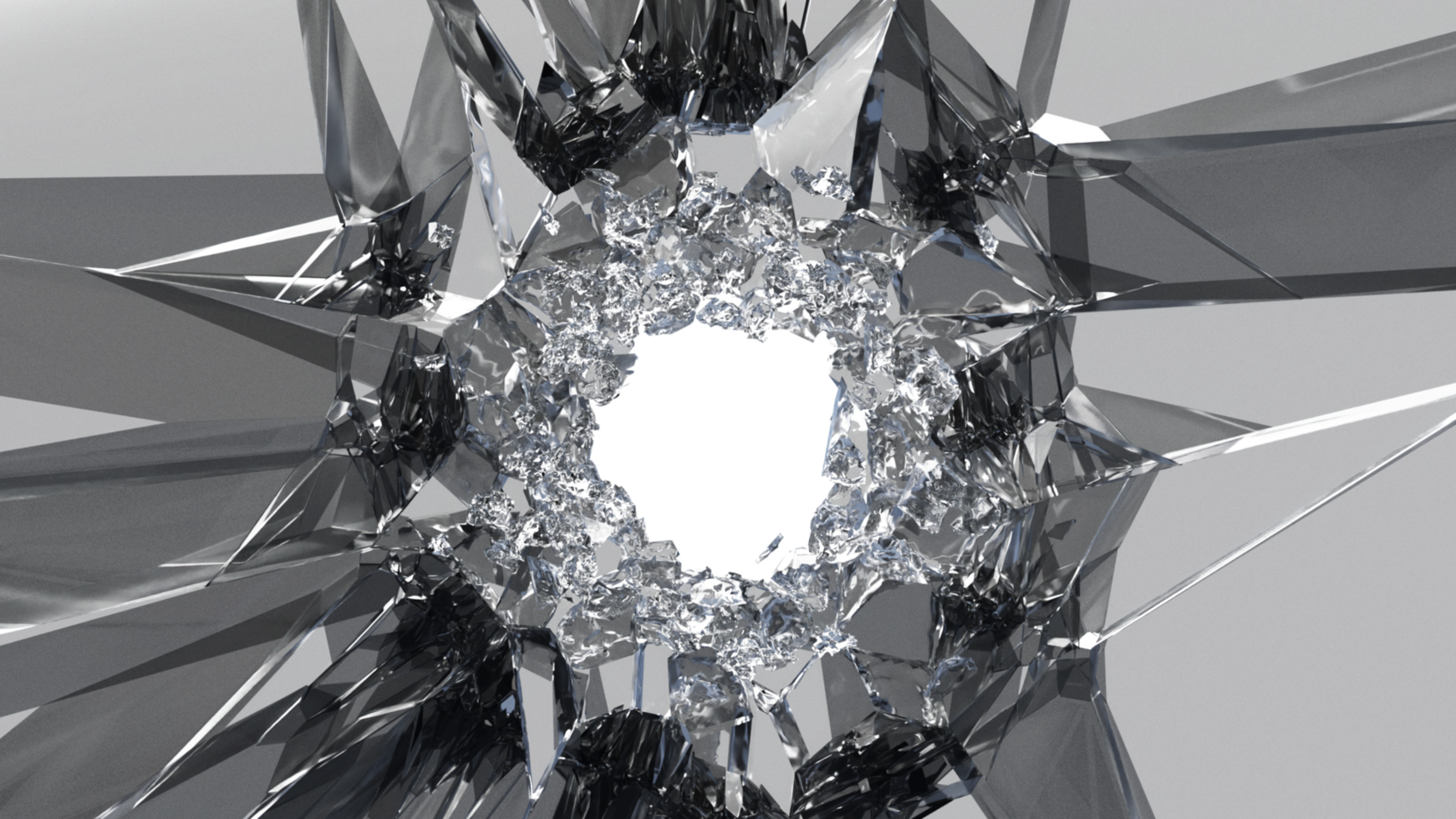The image is a black and white photograph of a crystal-like figure that appears to have been shattered. This intricate piece features a multitude of sharp, glass-like shards or spikes radiating outwards in every direction, giving it a jagged and fragmented look. The shards, varying in size, exhibit a mix of translucent and reflective surfaces that resemble either glass or metal. At the very center of this structure, there is a hollowed-out portion that is completely white, giving a stark contrast to the rest of the image. Surrounding this central white area are what appear to be crushed or crumpled aluminum foil-like elements, enhancing the fragmented and broken appearance. The background of the image is a medium gray, which helps to further highlight the complex, shiny, and sharp characteristics of the shattered crystal object.